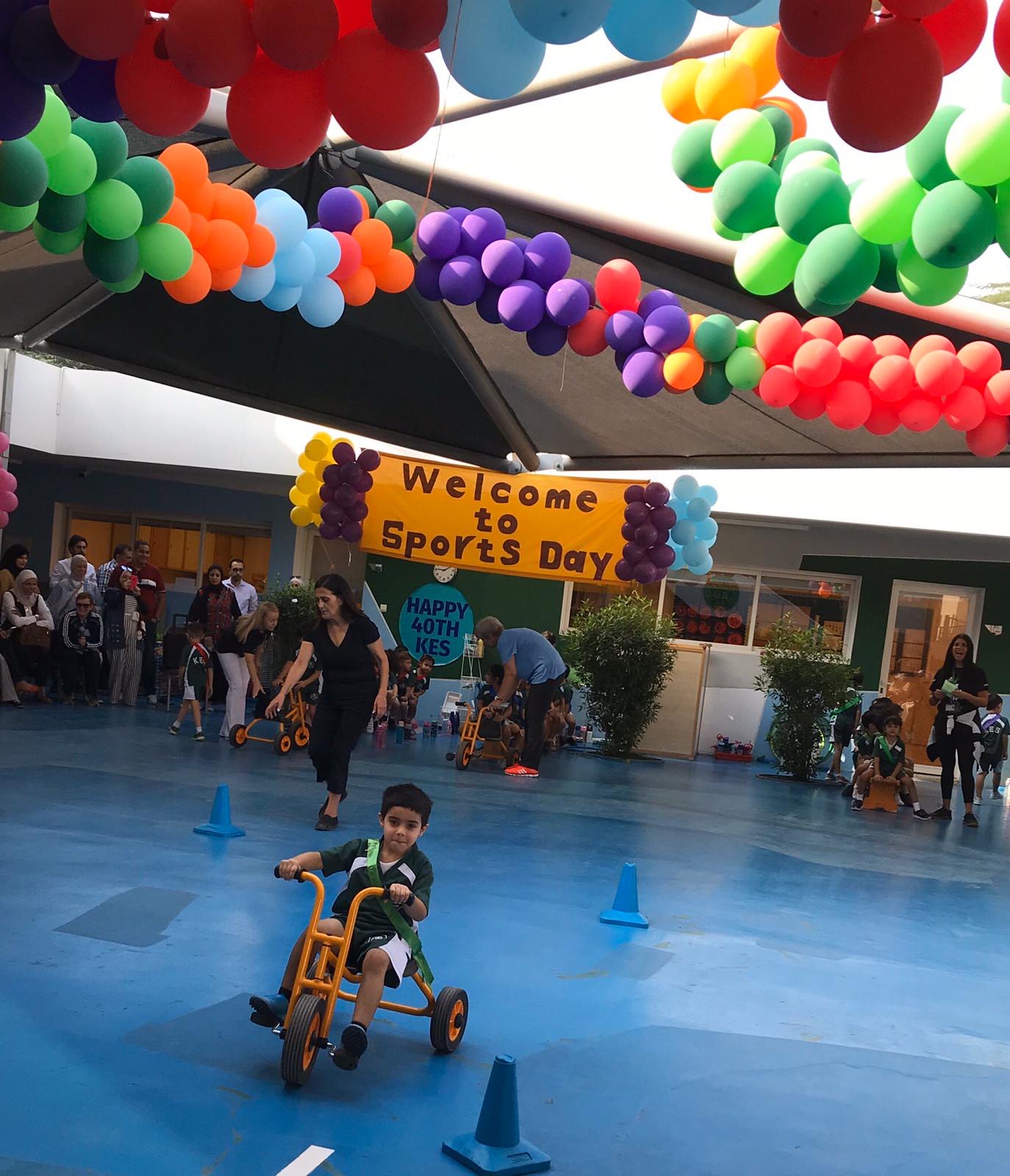The image captures a lively indoor event titled "Welcome to Sports Day," celebrating the 40th anniversary of KES. The scene includes a large yellow banner adorned with colorful balloons—red, blue, green, yellow, purple, and orange—welcoming participants to the sports day. Below the banner is a blue circle with the text "Happy 40th KES." There are windows and a door in the background, with some bushes visible outside. 

In the foreground, a young boy, around 2 to 5 years old, rides a yellow tricycle, navigating through blue cones on a blue floor, part of an obstacle course. He has dark hair and is dressed in a dark green shirt and shorts with white accents. Nearby, a woman with dark hair, dressed in a black shirt and pants, walks towards a cone. 

The background is bustling with activity, showing numerous adults, likely parents, and children either on tricycles or standing around. Some older adults can be seen to the left. The decoration features balloons hanging from the ceiling, creating a festive atmosphere that complements what appears to be a jubilant celebration of community and fun.